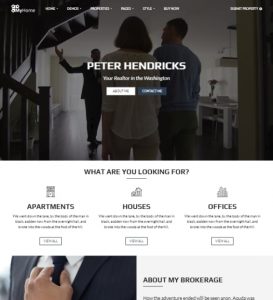The image showcases a real estate website interface. At the top, there's a blurry menu with various clickable options. The main picture below this depicts a bright, sunlit room in a home. Large windows flood the space with natural light. On the left side of the room, a staircase curves gracefully upwards. On the right, a table with a lamp adds a touch of hominess. In the center of the room, three people are present—one man in a suit and a casually dressed man and woman—potential buyers inspecting the house.

Text overlays in the image include the name "Peter Hendricks" followed by two clickable boxes: a white one on the left and a blue one on the right. Below this, a query reads, "What are you looking for?" with options for "apartments," "houses," and "offices," each accompanied by a descriptive paragraph and a selectable button. At the bottom, an advertisement titled "About My Brokerage" features an image of a person adjusting their necktie, suggesting professionalism and readiness to assist clients.